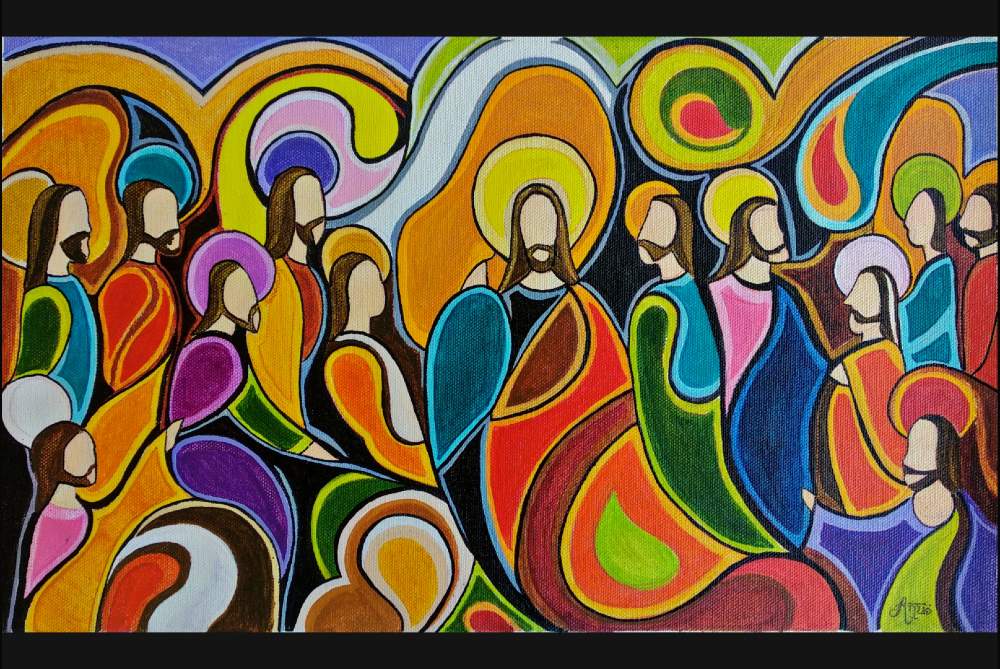This horizontally aligned rectangular painting, framed with thick black borders on the top and bottom, is a vibrant and abstract rendition of the Last Supper. The central figure, identifiable by his long brown hair and facial hair, resembles Jesus, with an array of overlapping, multicolored gowns surrounding him. These vibrant hues, including orange, yellow, pink, blue, green, red, purple, teal, fuchsia, and neon green, form swirling patterns and teardrop shapes between approximately 20 heads, all facing different directions. The figures alongside, likely representing the twelve apostles, also feature diverse facial hair, enhancing the textured appearance of the canvas. The signature in the lower right corner adds a final touch of authenticity to this colorful, psychedelic, and religiously iconic artwork.